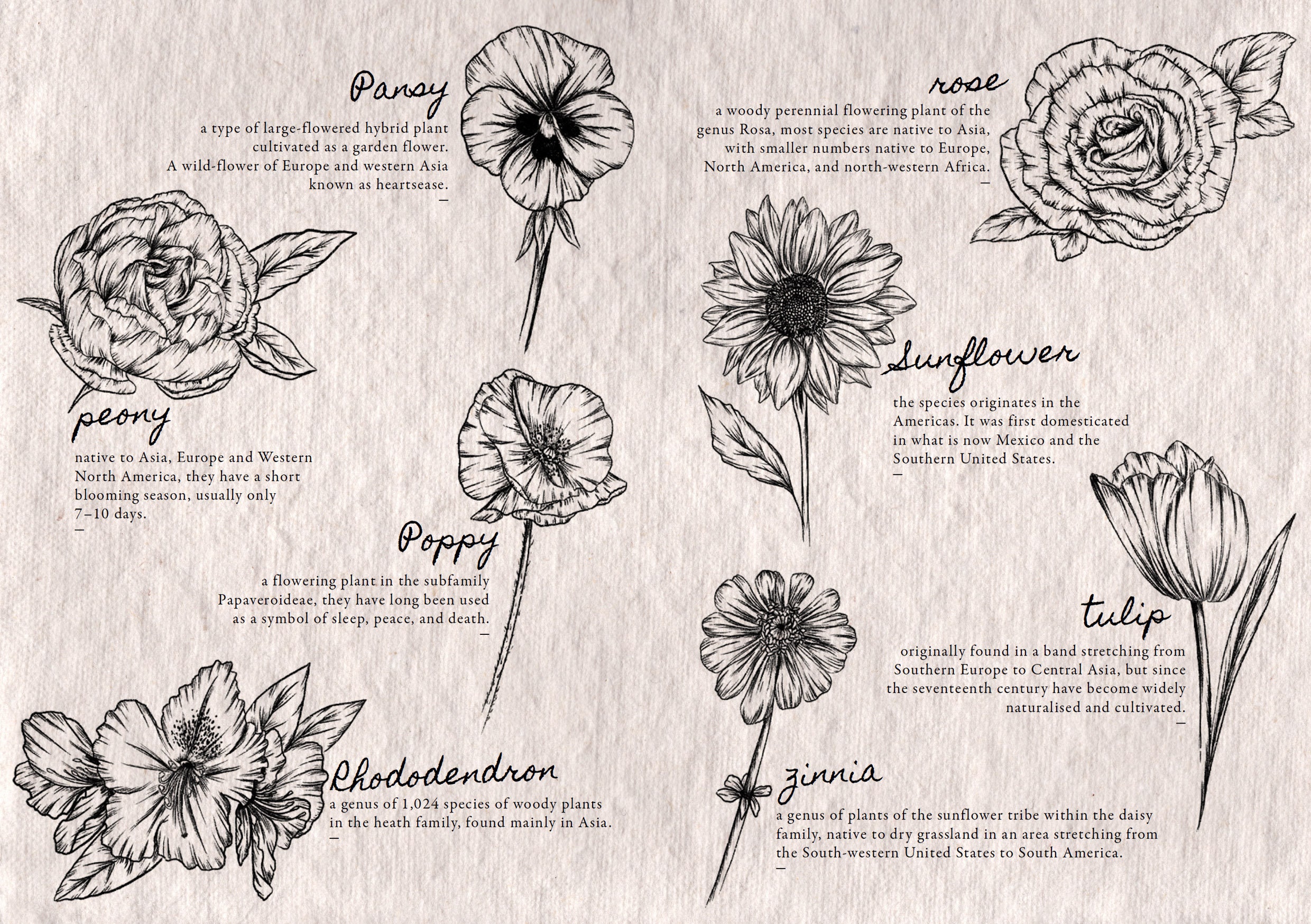The image is a digitally stylized guide to basic flowers, featuring detailed black-and-white illustrations of various flower species on a textured, fibrous white background resembling coarse paper. In a landscape orientation, each flower is presented on this page with its name written in cursive, followed by a concise description in black print. On the left side, the flowers listed include:
- **Pansy**: A large hybrid plant cultivated as a garden flower, native to Europe and Western Asia, commonly known as hearts ease.
- **Peony**: Native to Asia, Europe, and Western North America, noted for its short blooming season of 7-10 days.
- **Poppy**: A plant within the subfamily Papaveroideae, historically symbolizing sleep, peace, and death.
- **Rhododendron**: Encompassing 1,024 species of woody plants in the Heath family, predominantly found in Asia.

On the right side, the flowers include:
- **Rose**: A woody perennial plant of the genus Rosa, with most species native to Asia and fewer species native to Europe, North America, and northwestern Africa.
- **Sunflower**: Originally from the Americas, first domesticated in regions now known as Mexico and the Southern United States.
- **Tulip**: Initially found in a band from southern Europe to Central Asia, becoming widely cultivated since the 17th century.
- **Zinnia**: Belonging to the sunflower tribe within the daisy family, native to dry grasslands stretching from the southwestern United States to South America.

This guide serves as an educational tool, featuring monochrome illustrations and textual descriptions to help users identify and learn about different flowers.